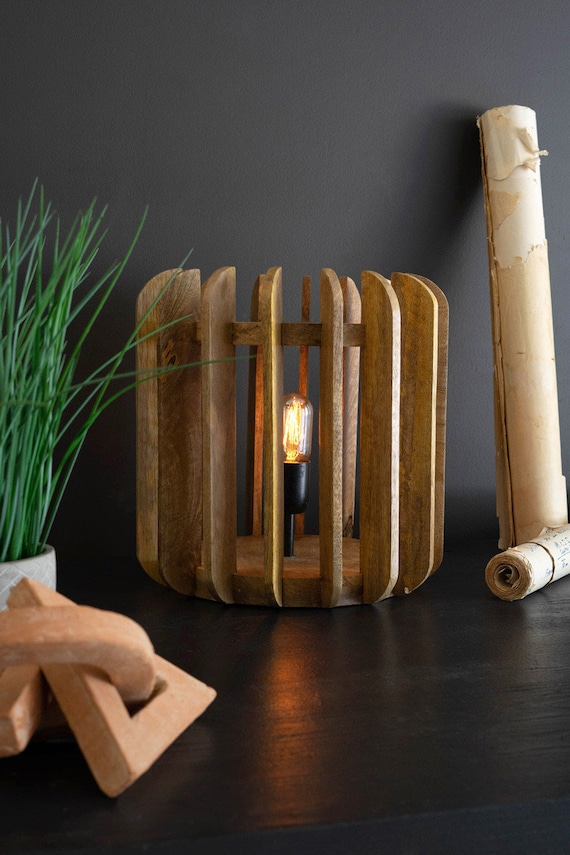The photograph showcases a meticulously crafted lamp composed of rounded wooden slats encircling a central Edison-style bulb. The bulb emits a warm, orange-yellow glow from its top and features a contrasting black base. The lamp is positioned on a gray wood table that adds a subtle rustic charm to the scene.

In the left foreground of the table, a wooden puzzle captivates the eye with its intricate interlocking circles and isosceles triangles, all made from a light, blonde wood. Just behind the puzzle, a white ceramic pot cradles a vibrant green chive plant, its slender leaves adding a touch of nature to the setting.

To the right of the lamp, a primitive-style musical instrument resembling a pipe is displayed with its lengthy shaft and a base designed for blowing, lending an artistic and eclectic touch to the arrangement. The entire setup is framed against a charcoal black wall, which accentuates the warm hues of the lamp and the natural tones of the wooden elements, creating a harmonious and visually engaging composition.